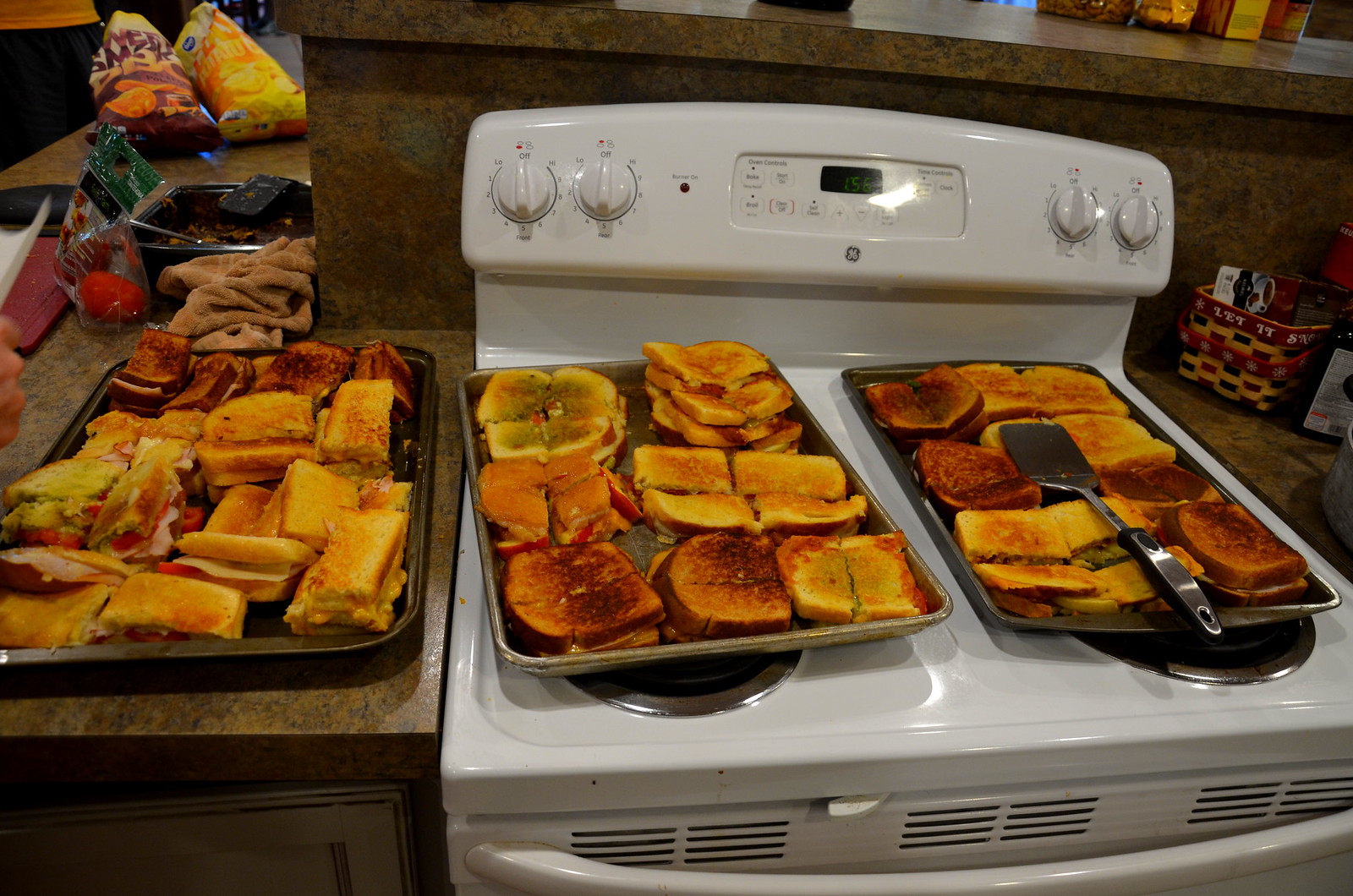This detailed kitchen scene depicts a white stovetop and oven combination set against a brownish marble countertop with subtle patterns. On the stove, filling its burners, are two trays laden with an assortment of grilled sandwiches. These sandwiches vary in type, with some showcasing the classic grilled cheese with their distinct melted yellow cheese and toasted golden-brown crusts, while others appear to contain different meats and fillings. A silver spatula rests atop one of the trays. To the immediate left of the stove, another greyish-brown tray holds more sandwiches, also cut up, probably prepared through a combination of baking and frying. Above this countertop area, two bags of potato chips are visible, adding a casual, hearty touch to the setting. 

On the right side of the image, adjacent to the stove, is the continuation of the brownish marble countertop featuring a red and yellow basket in the corner. The countertop has a lip that slightly juts out above the stove. In the background, a metal tray filled with some dark food can be seen along with some colorful bags of bell peppers. The kitchen embodies a bustling, somewhat cluttered atmosphere, as if in the midst of preparing a hearty meal or perhaps feeding a small crowd. The control panel on the stove features four white knobs and a center display with green numbers on a black background, though the time is indiscernible. Towels and other miscellaneous items complete this vividly detailed culinary snapshot.